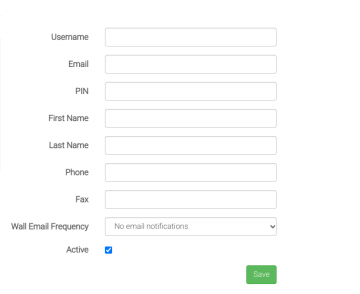This form allows you to input various personal details, including your username, email address, PIN, first name, last name, phone number, fax number, and email frequency preferences. Additionally, there's a section where you can indicate your active status. Although I'm not entirely sure of the form's specific purpose or the website it's from, these fields are present. Once all the necessary information is filled in, you can click the prominent green 'Save' button to submit the form.